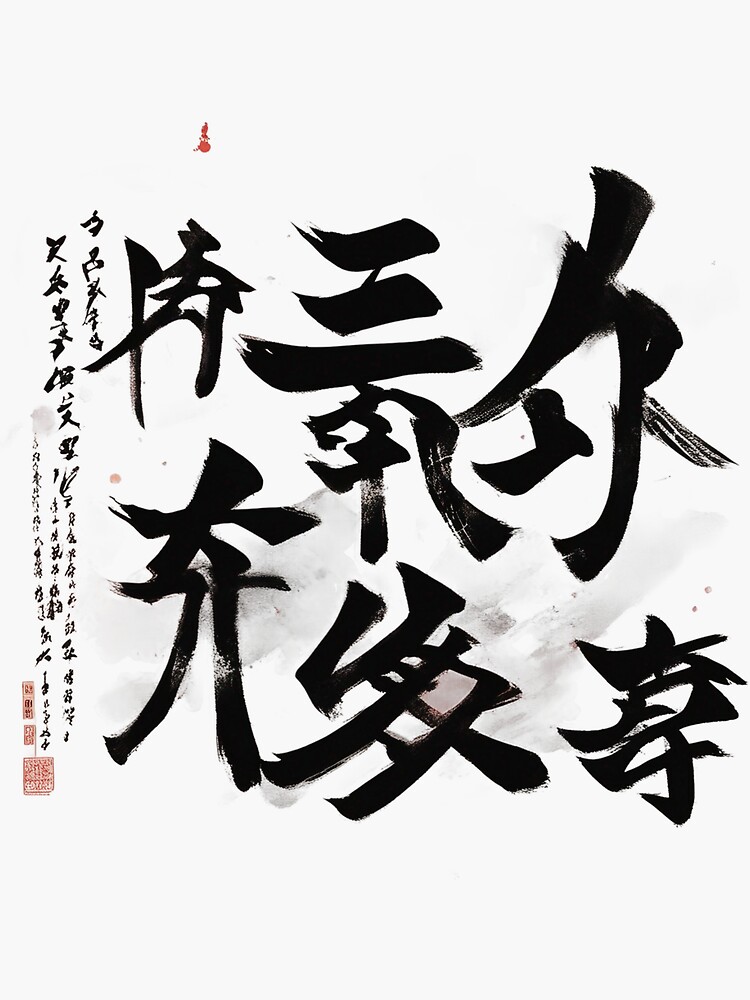This image features a piece of white paper with extensive Japanese text, depicted primarily in bold black ink. Dominating the top and bottom of the paper are six large Japanese characters, three at the top and three at the bottom, hastily written and slightly smeared, suggesting a quick or informal writing style. To the left, there are four columns of smaller, vertical black text. In the middle-left of the page, red ink appears in splotches and smaller symbols, including some that don’t resemble traditional kanji. At the very bottom left, there are three patterned red boxes—perhaps denoting a QR code or another form of information. The only colors in the image are the black ink of the characters and the vibrant red splotches, standing out starkly against the white background.